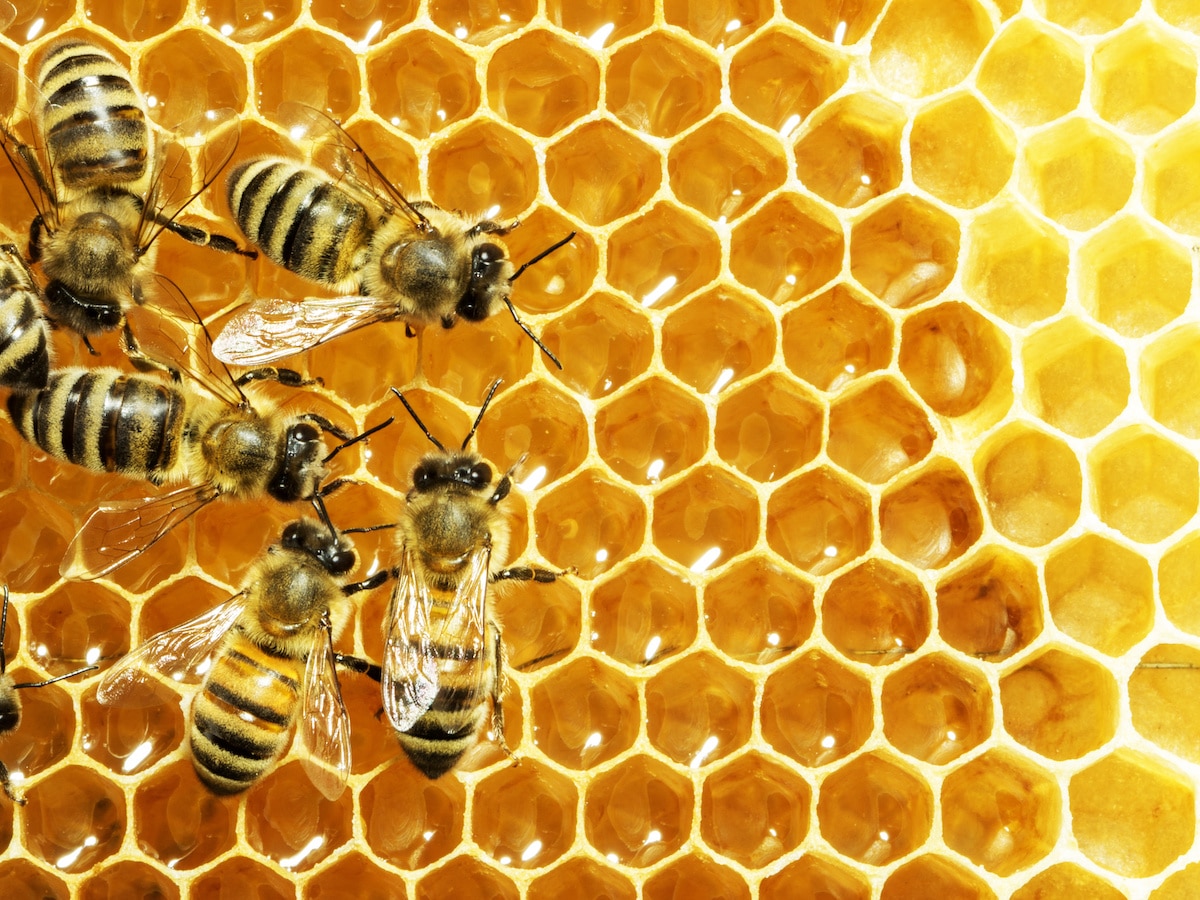This close-up photograph captures six bees on a vibrant honeycomb. The honeycomb, bathed in hues ranging from deep yellow to a beautiful orange-yellow, is laden with glistening honey, particularly on the left side of the image where the bees congregate. The composition shows five fully visible bees and the tail end of another, all of which appear to be feeding. The topmost bee in the left corner faces downward, while the two beneath it face rightwards, and the two below them look upwards. The right side of the honeycomb shows some cells yet to be filled with honey. The image, taken from an overhead angle, offers a detailed view of the bees and the intricate structure of the honeycomb, emphasizing the natural beauty and symmetrical patterns found within a beehive.